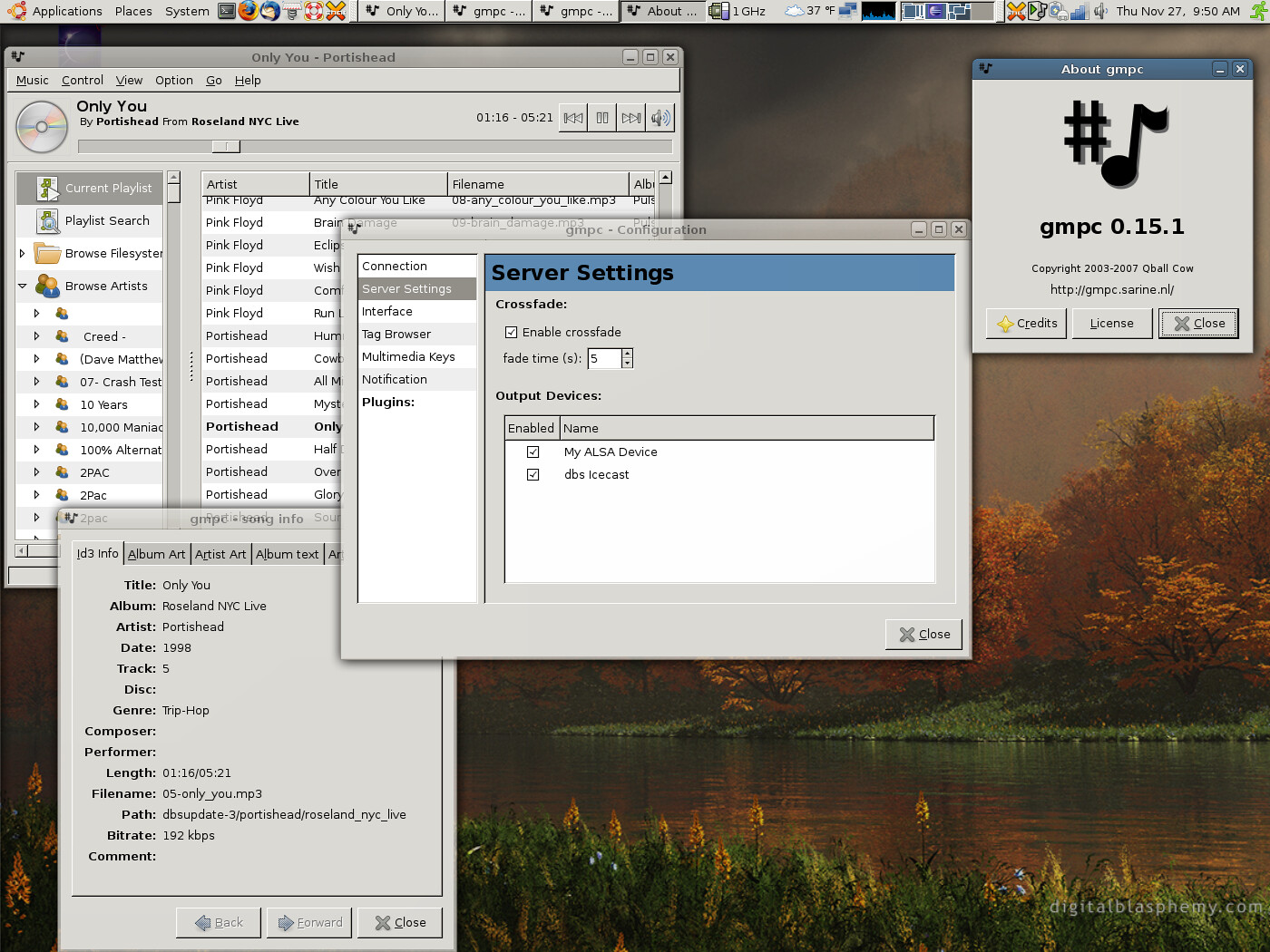The photograph captures an old computer screen displaying a variety of gray windows with thin gray tops, featuring black text and interactive buttons. The unusual aspect of the desktop is the taskbar positioned at the top of the screen instead of the bottom. This taskbar shows applications, places, system options, several icons, and the date and time—Thursday, November 27th at either 8:50 or 9:50 a.m., with the temperature reading 37 degrees F. The background image on the desktop is an autumnal photograph of a peaceful creek, bordered by grassy fields and trees adorned with yellow leaves.

Four distinct windows are open, each varying in size and location. Dominating the center is a window titled "Server Settings," displaying sections such as connection, server settings, interface, tag browser, multimedia keys, notifications, plugins, my ALSA device, and DBS IceCast. To the right, there's another window labeled "About GMPC" featuring a music symbol. In the upper left, a window with the title "Only U. Portishead" indicates music is being played. Finally, a smaller window at the lower left shows information related to music, including details about the artist and album. The overall setup suggests the user is managing a server and listening to music simultaneously.